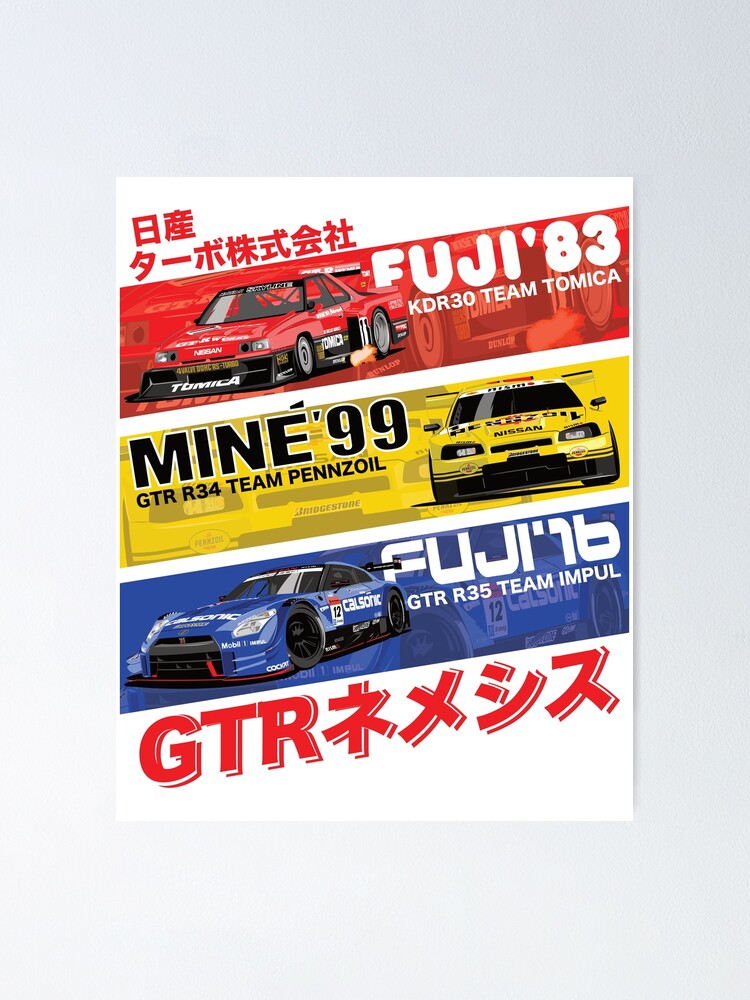The poster is a colorful advertisement for an auto racing event featuring Japanese text and detailing three different race cars. Each race car is displayed in a horizontal band with distinct colors: a red band, a yellow band, and a blue band. The top band is red and features a red Nissan car with the text "Fuji 83 KDR 30 Team Tomica." Above this band, there's additional Japanese text. The middle band is yellow and showcases a yellow Nissan race car with the text "Mine 99 GTR R34 Team Pennzoil." The bottom band is blue and depicts a blue Nissan race car with the text "Fuji 76 GTR R35 Team Impul." The car also bears the branding "CalSonic." At the very bottom of the poster, outside the color bands, it says "GTR" in red lettering followed by Japanese characters, reinforcing the theme of a racing event.